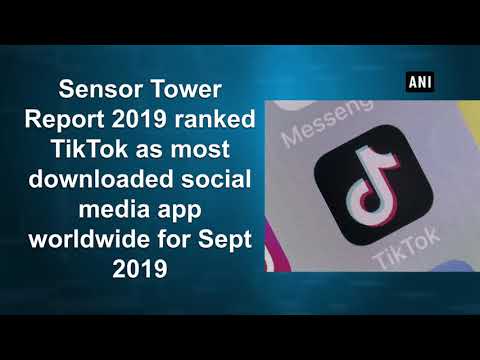The image appears to be an advertisement pop-up with distinct borders and information regarding a report. The top and bottom borders of the advertisement are black. The central section features a teal background.

On the left side of the advertisement, the text is written in white. The top line reads "Censor Tower," with each word beginning with a capital letter. The subsequent line says "Report 2019 Ranked," where "Report" starts with a capital "R." Below that is the word "TikTok," with both "T"s capitalized. The next lines read "Downloaded Social Media App Worldwide," where "Worldwide" is written as a single word. Following that is the abbreviation "SEPT" for September, written in capital letters, and the year "2019" is placed below it.

On the right side of the advertisement, there is a black rectangle with bold white letters that spell "A-N-I." Adjacent to this rectangle is a larger, predominantly black rectangle containing a black square within it. The square features the TikTok symbol, resembling a musical note. Below this symbol is the word "TikTok." Above the symbol, part of the word "messenger" is visible, although the "G" is partially cut off and the "E-R" is not visible at all.